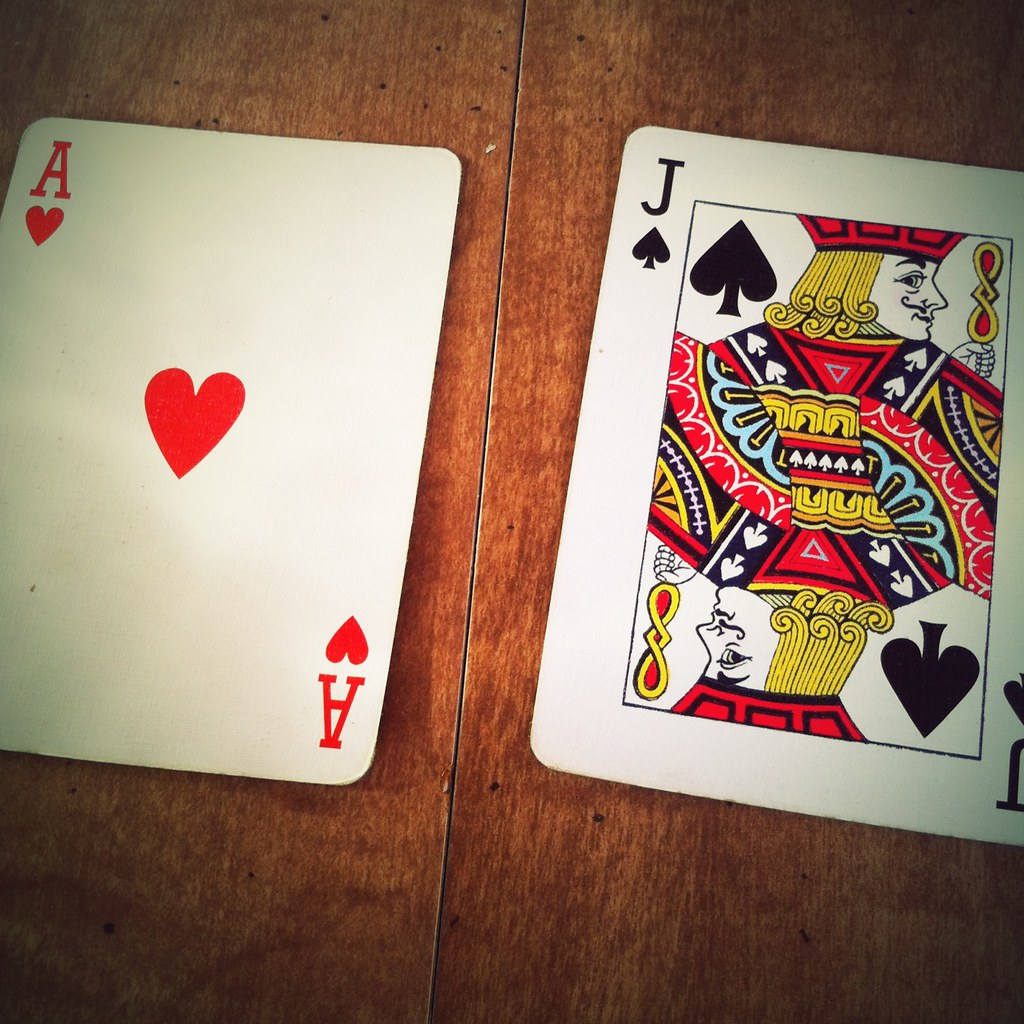The image depicts two playing cards placed on a dark hazelnut-colored wooden table. On the left, there is the Ace of Hearts, characterized by its vibrant red heart symbol. To the right, there is the Jack of Spades, distinguishable by its ornate black detailing. The wooden table features a central seam that runs directly between the two cards. The photograph has a shadowy vignette effect, with dark corners that frame and focus the viewer’s attention towards the center, where the cards are positioned.